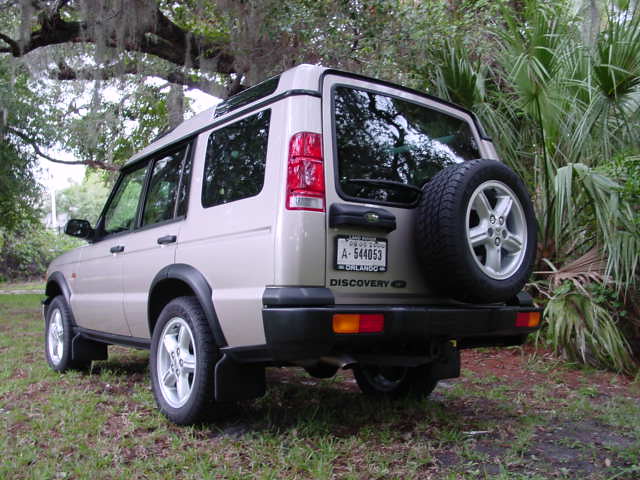The color photograph, taken outdoors on a bright sunny day, captures a brand new, beige Discovery model SUV parked on a grassy area adorned with semi-tropical greenery. The image is in landscape orientation, focusing on the rear and left side of the vehicle. This sporty, rectangular-shaped SUV boasts a spare tire mounted on its back door. A white dealer tag, framed with the word "Orlando," is visible, suggesting a Florida locale. The background is rich with verdant details, including patches of grass, brown dirt, palm fronds, leafy bushes, and an overarching tree with Spanish moss hanging from its branches. Light dramatically reflects off the vehicle's windows, emphasizing its newness and the bright, white skies overhead.